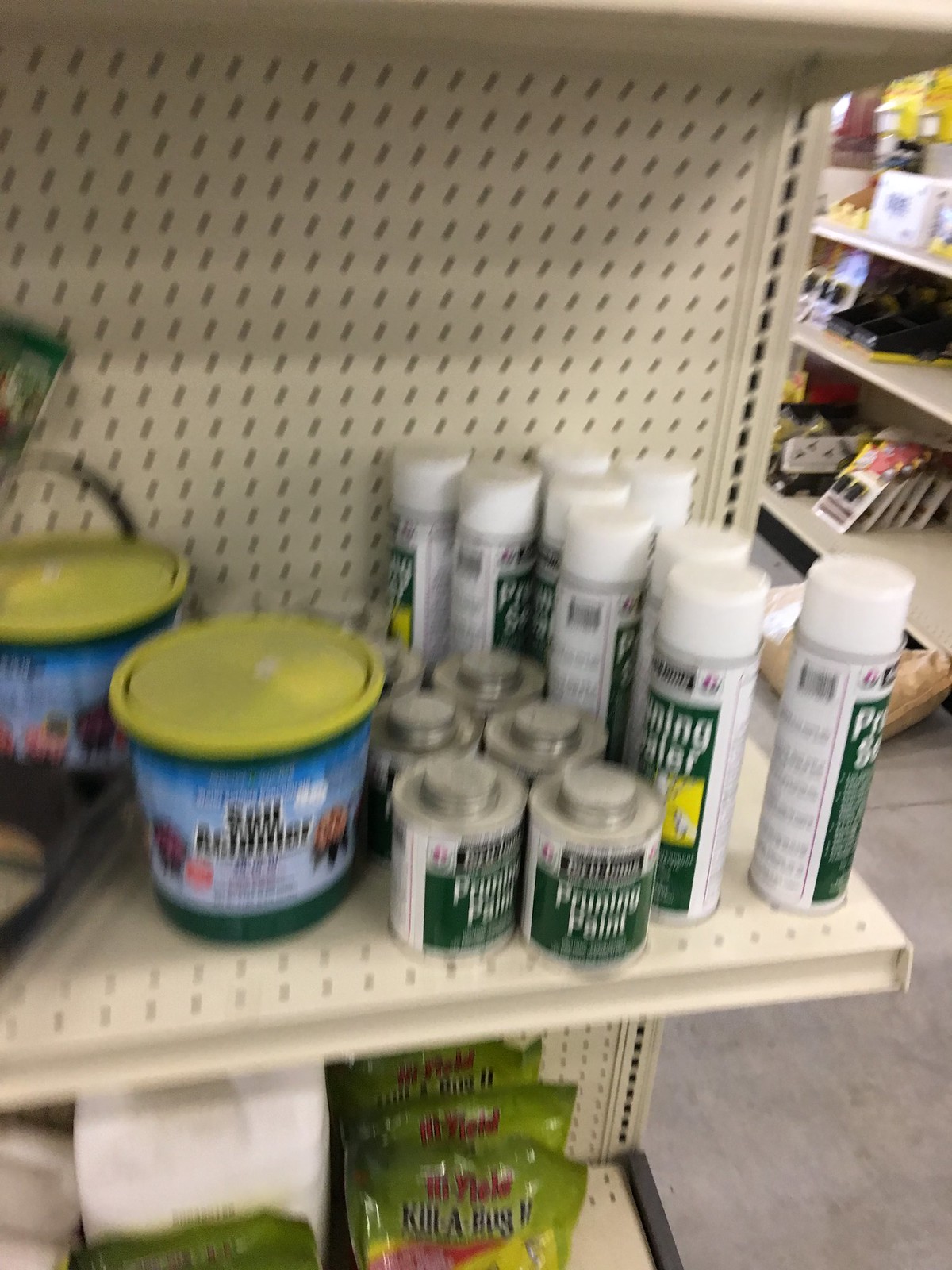A variety of products are displayed prominently on an end cap shelf in a hardware store. Despite the image being slightly blurry, one of the cans is labeled "Soil Acamide," another is labeled "Pruning Paint," and below, there is a product called "Kill a Bug." The setup suggests this is a convenient grab-and-go section for popular items, strategically placed at the center of the aisle. The larger aisle in the background indicates that this is indeed a hardware store, cemented by the concrete flooring typical of such establishments. The array of items suggests a focus on outdoor project supplies.